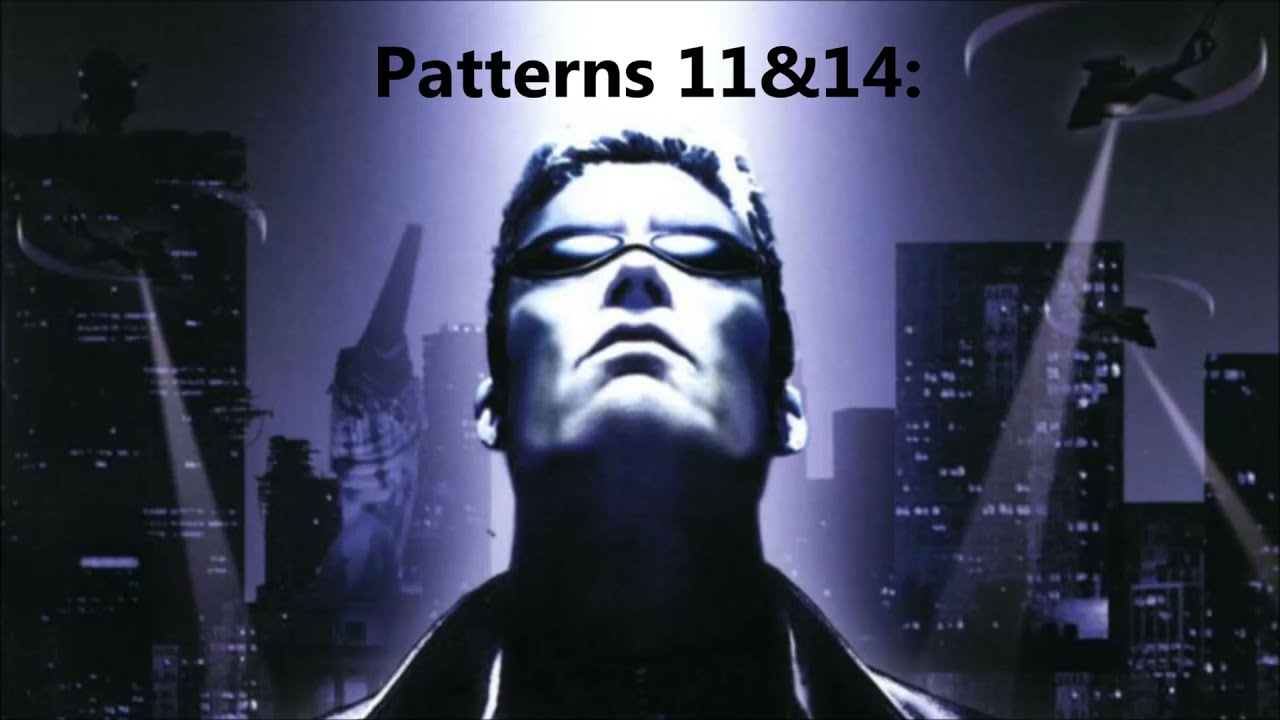The image depicts a man wearing small sunglasses, reminiscent of those seen in the movie "The Matrix," gazing upwards into the night sky. He stands front and center against a cityscape backdrop featuring five illuminated skyscrapers and a construction crane. The backdrop is dominated by shades of purple, black, and gray, with the man rendered in black and white. To the right and left above him, several UFOs hover, casting white beams of light downwards. The scene is bathed in a purplish hue. At the top center of the image, black text reads "patterns 11 & 14:". The intricate details and dramatic lighting suggest that this image might be an album cover or a movie poster.